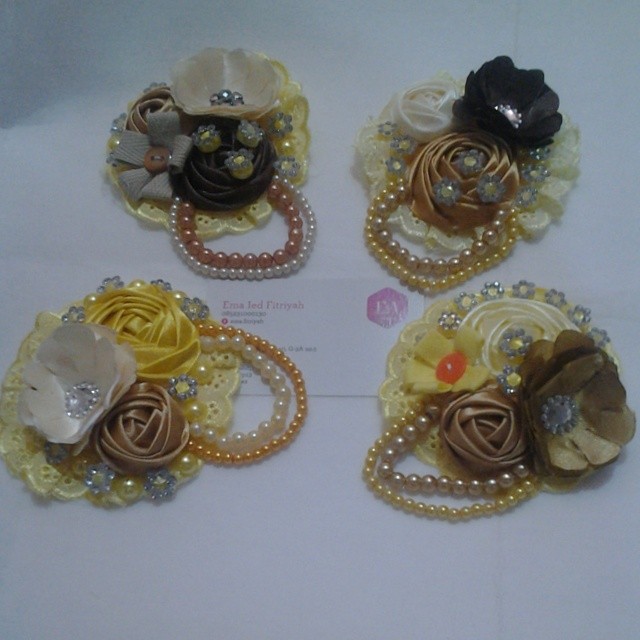The image showcases four fabric-crafted corsages arranged in a circular pattern around a partially obscured business card on a white background. Each corsage consists of a decorative doily base in light yellow and ivory tones, adorned with delicate beading in shades of lustrous pearl, light brown, and metallic hues. The beading forms two elasticated rings designed to wrap around the wrist, with finer beads on the outer ring and larger beads on the inner ring. Each corsage features a unique floral design: the bottom right one with four flowers, the bottom left with three, and the top two with similar floral embellishments. The flowers, made from various fabrics and materials, include grey fabric petals with brown button centers, designs simulating roses and rose buds, and ornaments with metallic balls and gray rhinestone petals. Amidst this intricately detailed display lies a business card, reading "Emma Led" with a purple hexagon logo partially visible, indicating the creator of these elegant, earth-toned ornamental pieces.